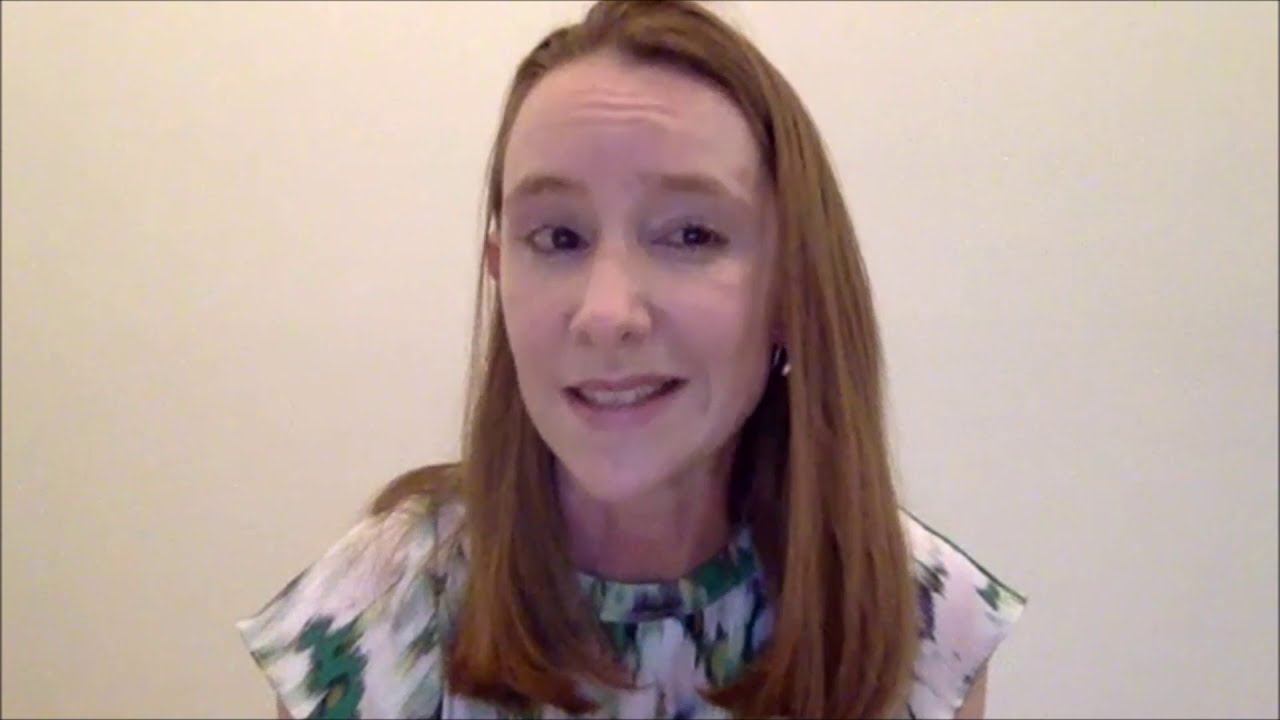In the image, a slender woman with shoulder-length, reddish-brown hair, possibly natural due to her matching eyebrows, stands out against a white wall background. Her hair, with a part on the right side, flows down to her chest, draped over both shoulders. She wears a short-sleeved, flowy floral top featuring greens, pinks, and whites. The woman, positioned centrally and viewed from the shoulders up, has a skeptical smile with three prominent wrinkles on her forehead, suggesting a mildly skeptical expression as if caught during a candid moment, possibly from an online video chat.